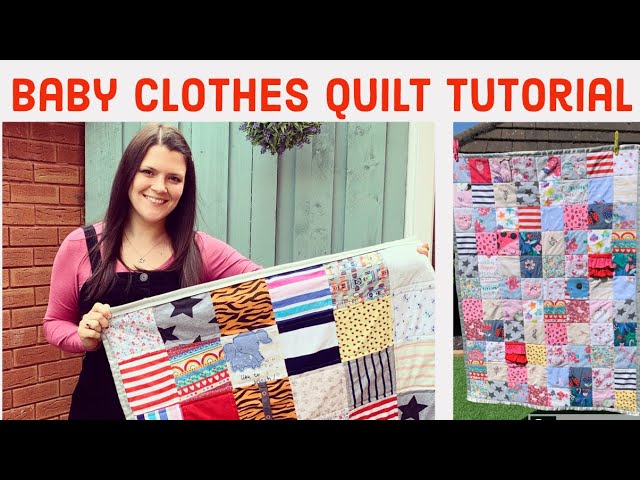The image features a tutorial for making a baby clothes quilt, prominently displayed with the text "Baby Clothes Quilt Tutorial" in red, all-caps, sans serif font on a white background near the top. Below the text are two photographs. On the left, a smiling young woman with long brown hair and light-colored skin is wearing a long-sleeved magenta shirt under dark black overalls. She stands in front of a red brick building with a white fence to her right and a flowering plant in the background, holding a patchwork quilt made from baby clothes, which includes squares with various prints such as animal patterns and stripes. On the right side of the image, a second photograph shows the entire colorful quilt, suspended from a clothesline, displaying its detailed, vibrant patchwork design.